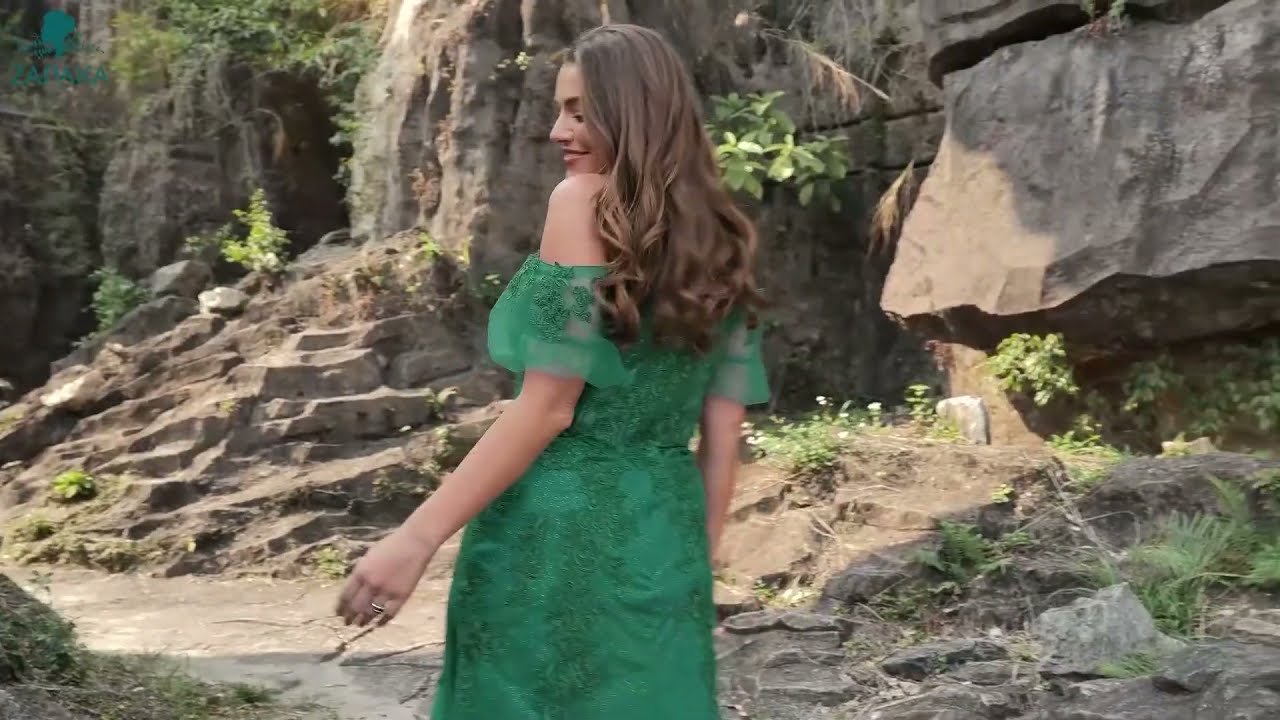The image captures a woman with light-tan skin and long, wavy brown hair that flows past her shoulders, wearing an elegant, off-shoulder emerald green dress adorned with the same colored embroidery. As she gazes over her left shoulder, a gentle smile graces her face, revealing her side profile. Her left hand, adorned with a wedding band and featuring red nail polish, is partially visible. She stands in a rugged, rocky area with brown stone cliffs and various greenery and shrub-like foliage growing in the cracks. The scene, bathed in natural daylight, features sunlight illuminating parts of the rock formations behind her, creating a serene, picturesque backdrop for this moment of quiet beauty.